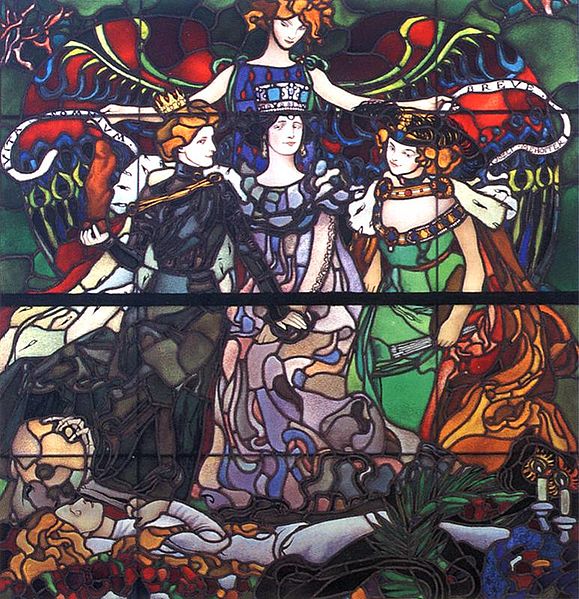This intricate stained glass window features a richly detailed scene set against a backdrop of vibrant and bold colors, reminiscent of the kind found in churches. The window is divided into numerous panels that seamlessly form a cohesive image. At the center stands a regal woman, likely a queen, adorned with a gem-studded crown and dressed in a multicolored ensemble of blues, whites, grays, and blacks. Her dark hair frames her face, accentuated by earrings, emphasizing her royal status. Flanking her are two additional women who also appear to be of noble standing, possibly queens themselves. The woman on the right wears a dark dress of blue hues and a golden, slightly tilted crown, while the woman on the left dons a green dress with an ornate headpiece.

Behind this queenly trio is a woman with wavy blonde hair, arms outstretched to display large, multicolored fans in shades of blue, orange, and yellow, adding a dynamic sense of movement and celebration. At the bottom of the window lies a prone woman with orangish hair, perhaps deceased, dressed in gray attire with a somber expression that suggests a funeral scene. Her hands are crossed over her chest, surrounded by lit candles at her feet, indicative of a commemorative rite. This striking portrayal, crafted from numerous pieces of glass, captures a poignant and dignified narrative, marrying sorrow and reverence in a bewitching tableau.